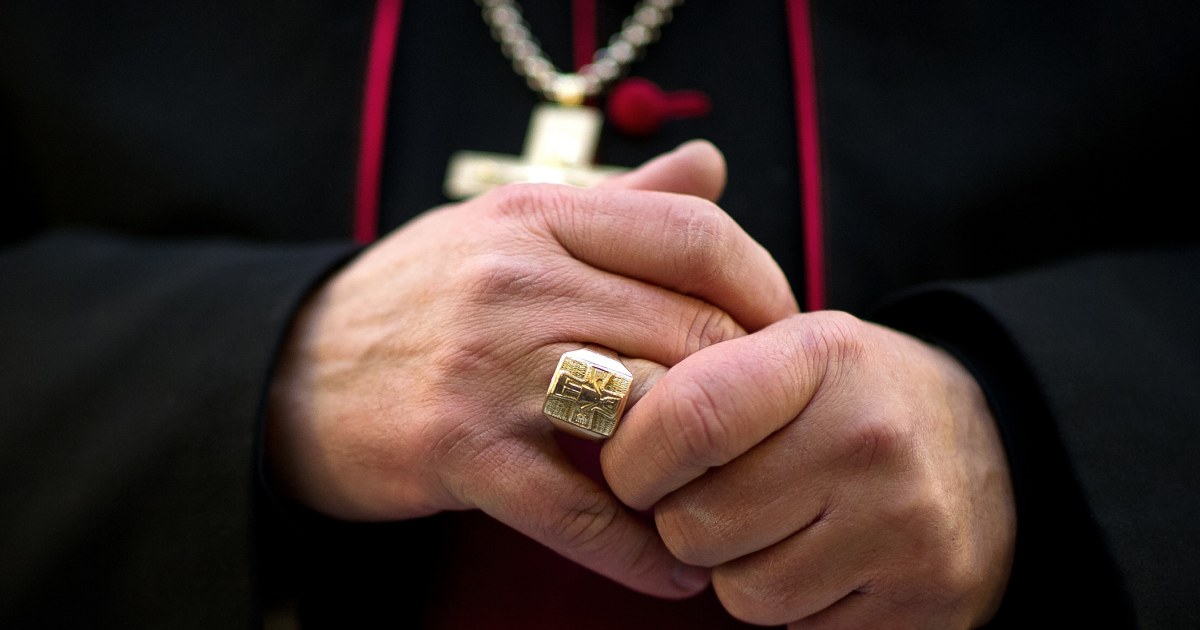The image is a close-up, landscape-oriented photograph capturing the detailed hands of a religious figure, likely a pope or bishop, wearing black robes—a cassock—adorned with prominent red stripes and numerous buttons. The focal point of the image is the clasped hands, which reveal the person’s pale, Caucasian skin, depicting fine wrinkles and pores in sharp detail. The right hand bears a significant golden ring on the ring finger, featuring a cross, known as the fisherman's ring, while the left hand appears to be adjusting or lightly holding the right ring finger. The gold cross on a chain around the neck partially spills into view, adding an element of grandeur. The blurred background emphasizes the detailed textures of the hands and the ornate elements of the religious garb, such as the black sleeves with cuffs extending to the wrists.